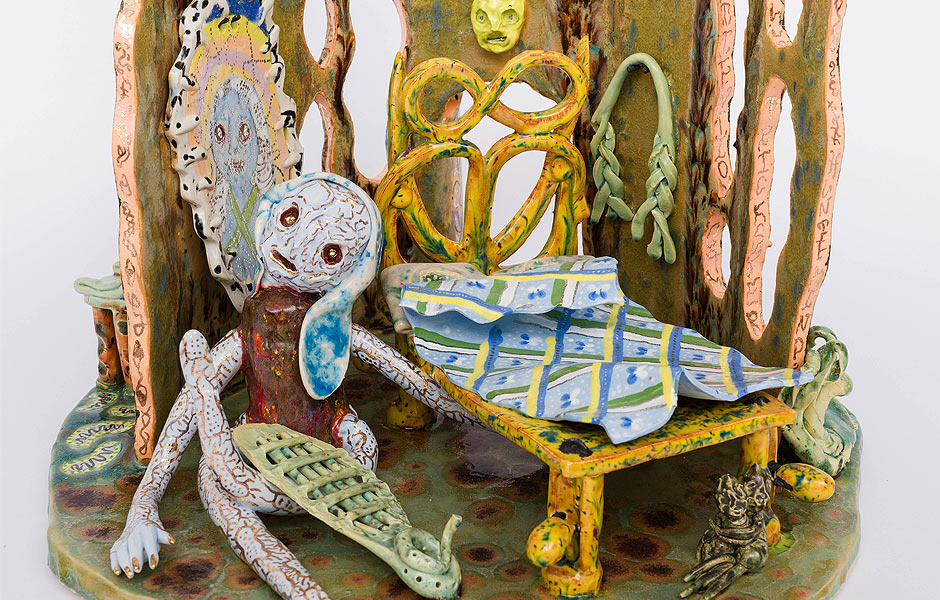The image portrays an eclectic art display on a uniquely patterned ceramic table. Central to the scene is a yellow bed, possibly crafted from metal or clay, with matching yellow legs. The bed is covered with a light blue blanket featuring plaid patterns of yellow and green lines, meticulously designed to mimic the appearance of a fold. Surrounding the bed are intriguing figures, including a person made from the same material as the bed, standing to its left, accompanied by an indistinct item. By the right leg of the bed, there are animals, though their exact nature is unclear. Above the bed, a face-like mask or image adorns the wall, adding an enigmatic touch. 

The entire display is set on a round, but not perfectly circular, platform. Around this platform stand three miniature gravestones, contributing to a conceptual vibe, possibly hinting at themes of sickness or disease as suggested by the predominantly brown and green color palette. On the floor, varied knickknacks include a rabbit-like statue with a peculiar paddle on its leg, a frog, a yellow stone, and a coiled body shape embedded in the bed’s headboard. Additionally, a braided rope is visible hanging on the wall, alongside what might be a painting or a mirror, completing this intricate and thought-provoking arrangement of art objects.